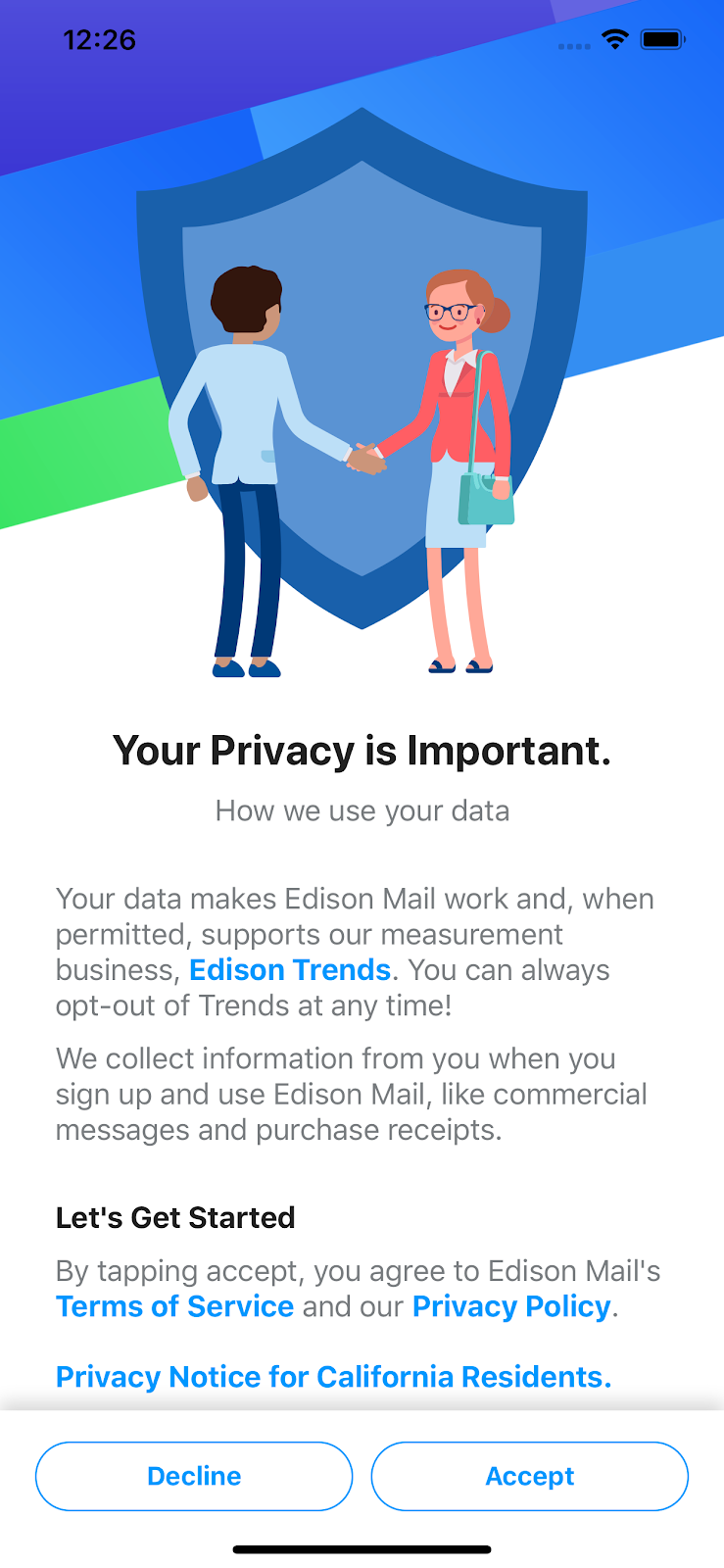The image depicts a web page, prominently featuring animated characters at the center. An African-American man wearing a light blue shirt, dark blue pants, and dark blue slippers is shown shaking hands with a Caucasian woman. The woman, who has brown hair tied in a ponytail, is dressed in a red dress over a gray undershirt and a light blue skirt, accessorized with a pair of blue spectacles, red lipstick, red earrings, and dark blue sandals. 

Behind the two characters is a shield outlined in dark blue, with a mid-blue center and a purple band at the top. The purple band includes the time "12:26" in a military format, ellipses, a full Wi-Fi signal symbol, and a fully charged battery icon, both in black. 

Below the animated characters, there is a text section starting with the bold, black headline: "Your privacy is important." This is followed by a gray text prompting, "How we use your data." The subsequent section states: "Your data makes Edison Mail work, and when permitted, supports our measurement business, Edison Trends. You can always opt-out of trends at any time!" 

Further down, another section explains: "We collect information from you when you sign up and use Edison Mail, like commercial messages and purchase receipts." Below this, the bold, black text says, "Let's get started." In gray text, it continues: "By tapping accept, you agree to Edison Mail's," followed by clickable blue text links to the "terms of service" and "Privacy Policy." There is also a clickable blue link for "Privacy notice for California residents."

At the bottom of the page, there are two oval buttons with dark blue borders: the left one labeled "Decline" and the right one labeled "Accept." The device's dark gray bezel and a black navigation bar are visible at the bottom of the screenshot.